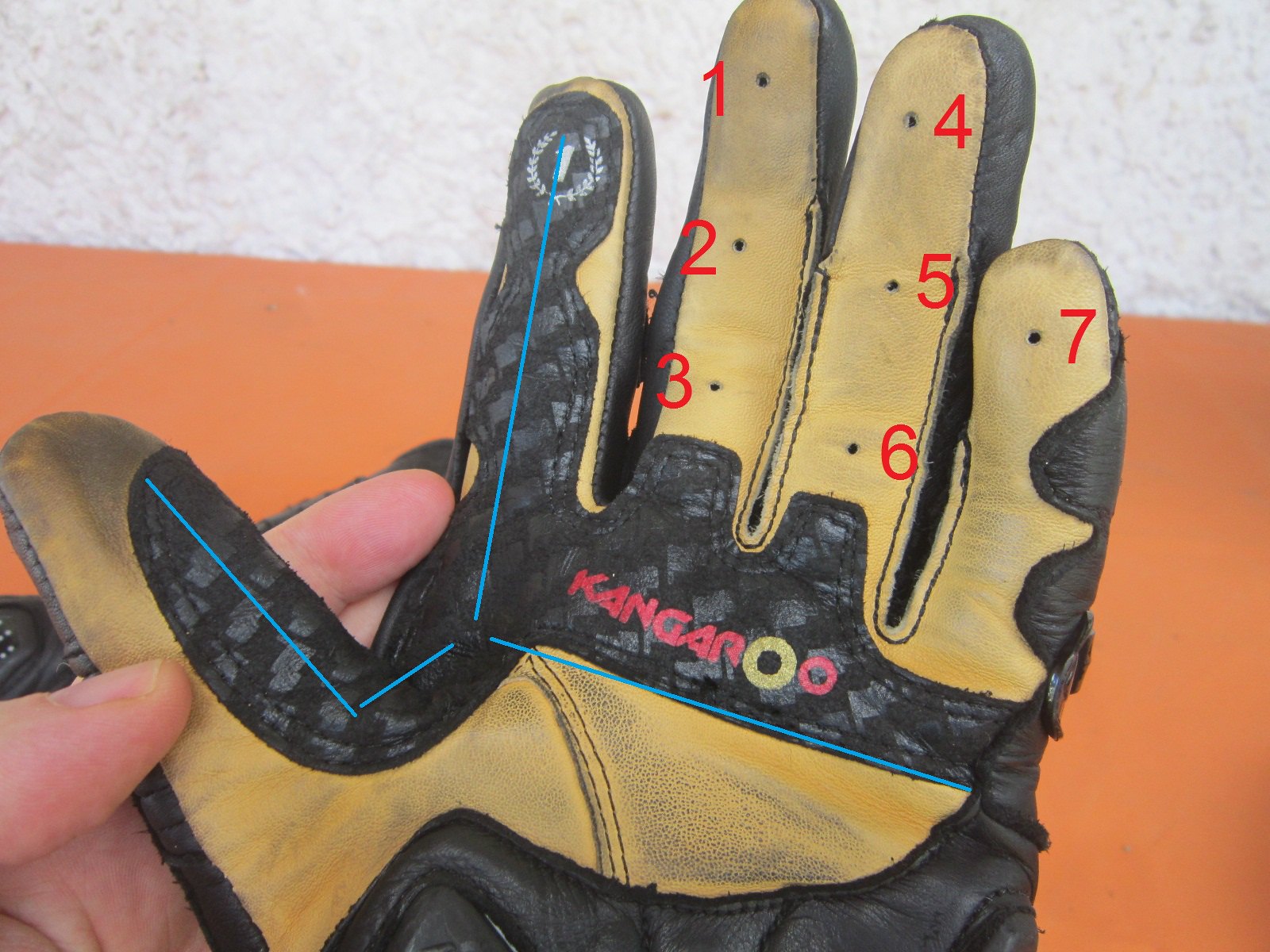This is a detailed close-up photograph of the palmar side of a used left-handed glove, prominently displayed against a background that is orange for the lower two-thirds and a white stucco material for the top third. The glove itself features a combination of black and yellow (or tan) leather. The black areas include the index finger, thumb, ball of the hand and edge of the pinkie, while the rest is yellow. The glove’s brand name, "Kangaroo", is printed on the palm in red text, with the first 'O' replaced by a larger yellow circle. A distinct feature of the glove is a white number '1' enclosed in an olive branch symbol on the tip of the index finger. Edited onto the image are thin blue lines that trace from the thumb to the pointer finger and across the palm. There are small holes punched through the leather on the fingertips of the middle, ring, and pinky fingers. Each hole is labeled with a red number, sequentially ranging from 1 to 7, with holes 1, 2, and 3 on the middle finger, 4, 5, and 6 on the ring finger, and 7 on the tip of the pinky. Blue informational lines and numbers suggest that the photo is intended to highlight specific features, possibly for a product listing or technical illustration. The picture also shows the thumb and fingers of the person holding the glove to the left side of the image.